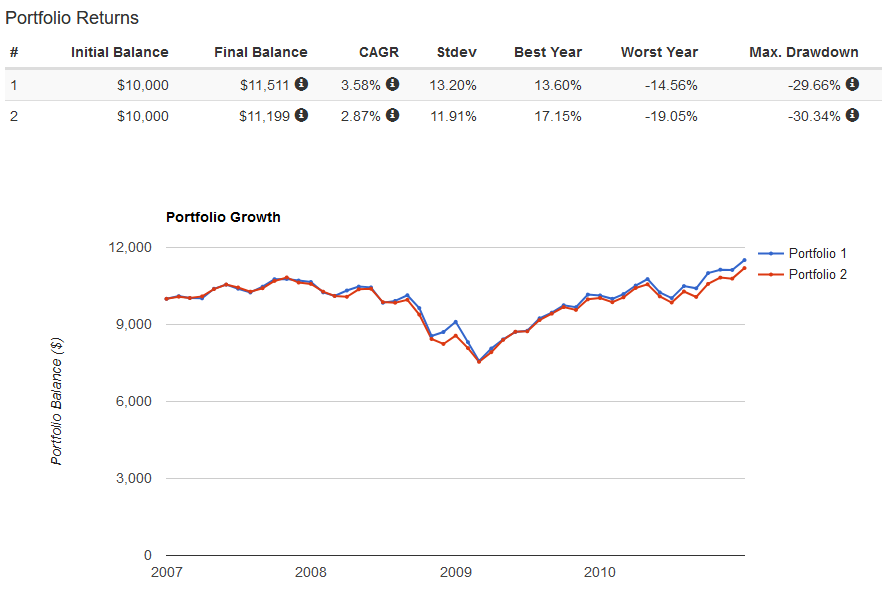The image is a detailed screenshot capturing portfolio returns on a white background. It comprises various financial metrics presented in a chart format, including symbols such as the Pound Sign (£), and data columns labeled: Initial Balance, Final Balance, CAGR (Compound Annual Growth Rate), STDEV (Standard Deviation), Best Year, Worst Year, and Max Drawdown. 

Under the Pound Sign identifier:
1. Portfolio 1 exhibits an initial balance of £10, which grows to a final balance of £1,511. The CAGR for this portfolio is 3.58%, with a standard deviation of 13.20%. The best year return is 13.60%, while the worst year shows a loss of -14.56%. The maximum drawdown recorded is -29.66%.

2. Portfolio 2 starts with an initial balance of £10,000, ending up at £11,199. The CAGR is noted to be 2.87%, accompanied by a standard deviation of 11.91%. This portfolio's best year performance is 17.51%, with the worst year declining by -19.05%. The max drawdown for Portfolio 2 stands at -30.34%.

The chart also contains an “i” in a circle, possibly indicating additional information or tooltip annotations. Additionally, the image depicts a portfolio growth graph at the bottom, spanning years from 2007 to 2010.